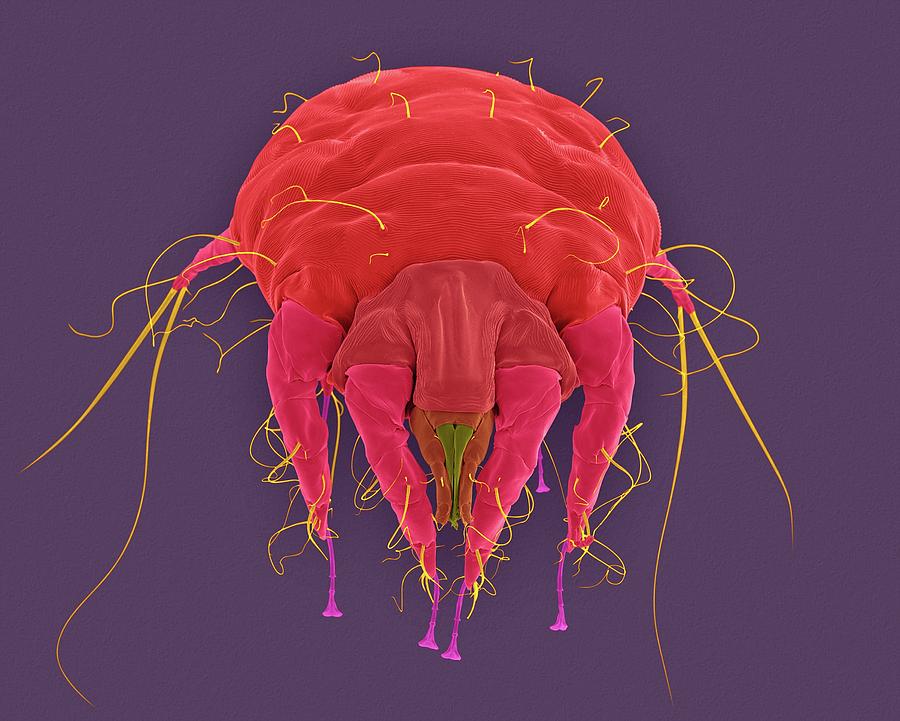This photograph showcases a close-up of a stuffed animal insect placed on a rich purple background. The insect's body is a vivid red, with four pink legs extended towards the front and two additional pink legs at the back. Sporadic yellow strands of hair emerge from its back, complemented by long yellow hairs extending from its sides and back legs. The creature features a distinctive mouth area, characterized by orange and green pinchers. Additionally, purple string is visible emerging from its hands and face, adding to its elaborate and whimsical design.